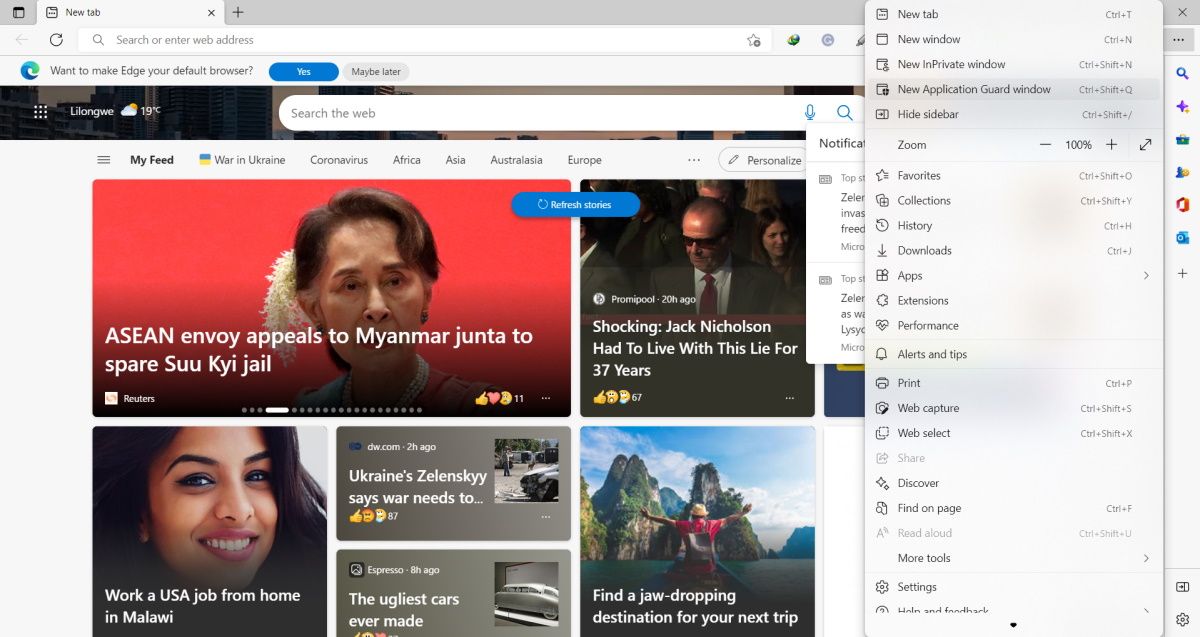An Edge browser window is shown open to the home page, which appears to be the typical MSN start page. Dominating the layout is a white, rounded search bar featuring blue icons for microphone input and a magnifying glass for text searches. The location is displayed as Lilongwe, with the temperature noted at 19 degrees Fahrenheit. Various headline stories populate the home page, focusing heavily on international news, including significant coverage of the war in Ukraine, prominent enough to be the top link in the user's feed. Other major topics follow, such as coronavirus updates and news from Africa, Asia, Australia, and Europe. A button labeled "Personalize" offers customization options for the news feed. Visually, the page is laid out in a grid format with images of various sizes. On the right side, an options menu is open, listing functions like opening a new tab, new window, new InPrivate window, zoom settings, and access to favorites, providing a comprehensive overview of available browser functionality.